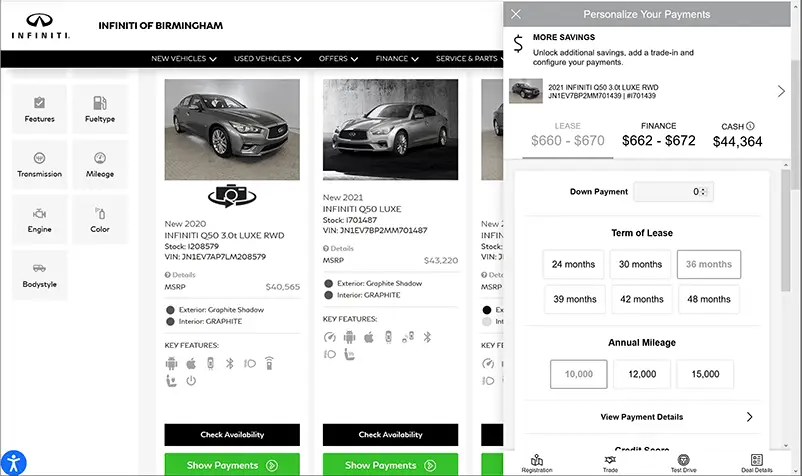This landscape-oriented screenshot showcases the official website for the car brand Infiniti, displayed in a format suitable for a computer or laptop screen. The interface includes a vertical pop-up column on the right side that partially obscures the main content. 

At the top of the page, a white header features the Infiniti logo along with the text "Infiniti of Birmingham". Below the header is a black, horizontally-aligned navigation bar with white text, offering drop-down menus for New Vehicles, Used Vehicles, Offers, Finance, Service, and Parts.

On the left side of the page, a white column contains several gray, clickable boxes labeled Features, Fuel Type, Transmission, Mileage, Engine, Color, and Body Style, allowing users to filter their search options.

The main content area displays vertically arranged white rectangular boxes, each presenting images and details of different car models. For example, the first listing features a "New 2020 Infiniti Q50", followed by a "New 2021 Infiniti Q50 Luxe". Each entry includes key descriptions, VIN numbers, and details on exterior and interior colors, represented with icons.

Additionally, each car listing offers a black, rectangular checkbox for selection and a green rectangular button labeled "Show Payments" for users to view payment options.